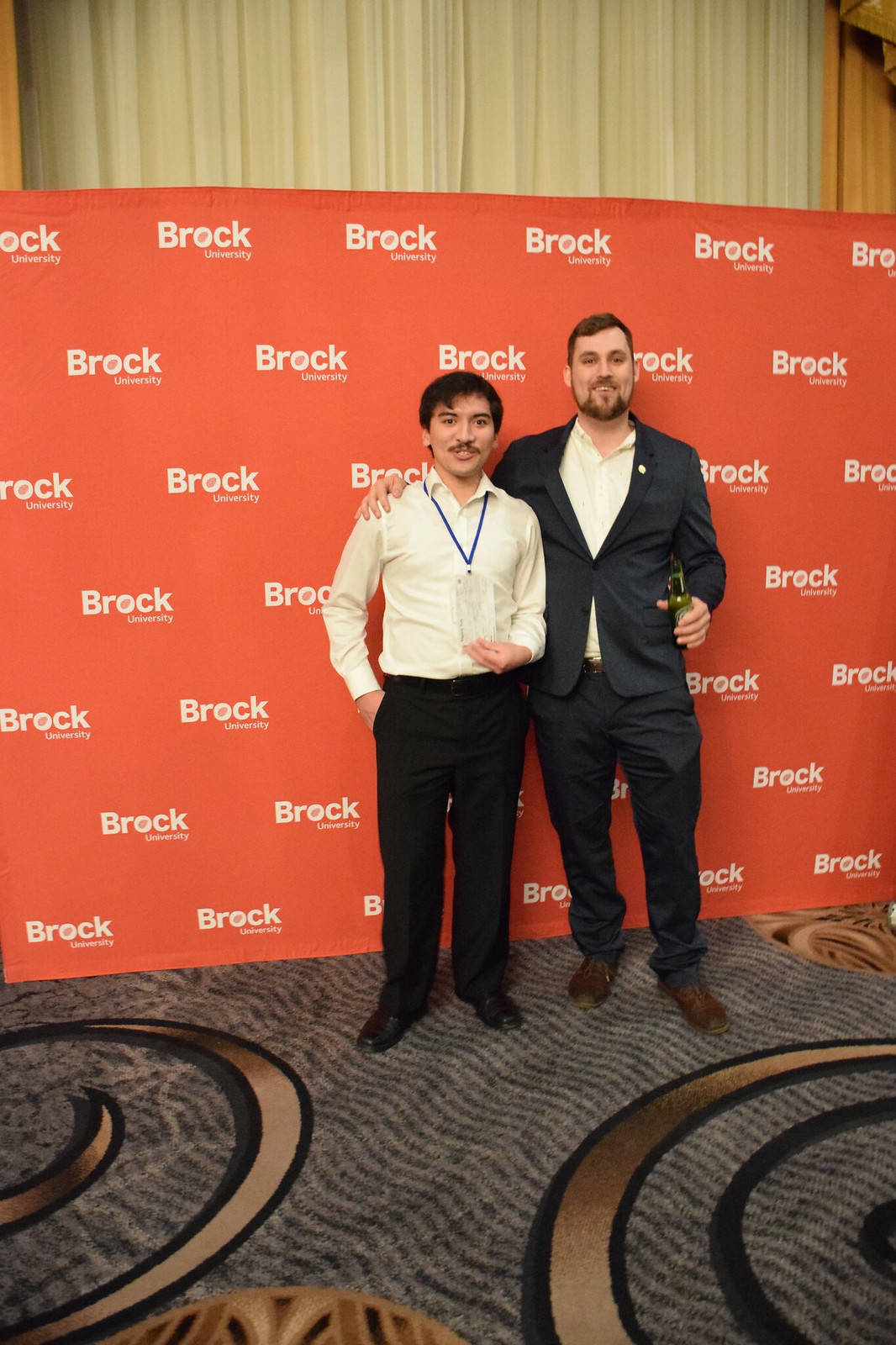This image captures two men standing on an intricately designed rug featuring a rich array of textures and colors including gold circles, black circles, and curly Q patterns on a grey and white striped background. Behind them, an orange wall prominently displays the words "Brock University" in white letters, with a cream-colored section above the orange backdrop. The man on the left is shorter, with a tan complexion, and sports a white dress shirt, a lanyard with a tag, dark pants, dark shoes, and has black hair and a mustache. The man on the right, taller and Caucasian, is dressed in a navy blue suit with a white shirt underneath. He has short brown hair, a beard, and is holding a green bottle of beer in his left hand. The two men, both smiling, appear to be at a professional event, perhaps a seminar or work gathering, creating an atmosphere of camaraderie and celebration.